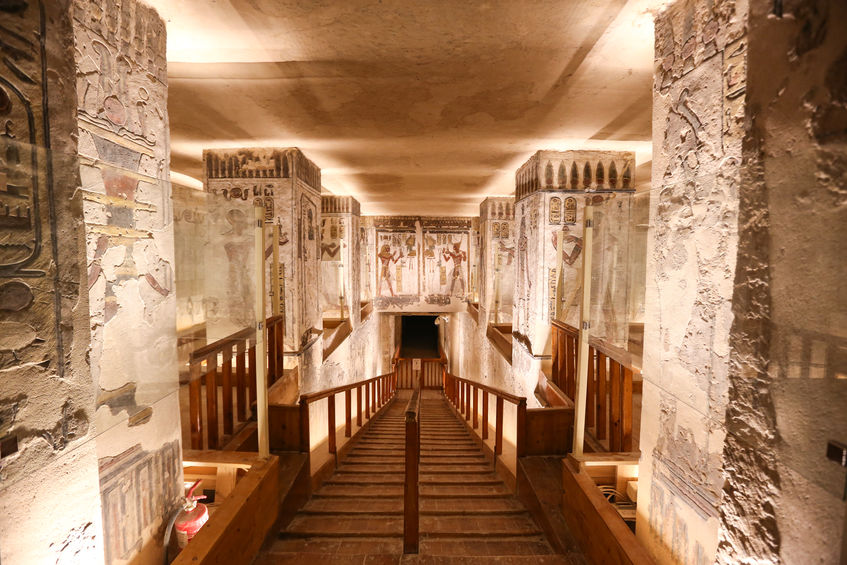The image depicts the interior of an ancient Egyptian museum or temple. The scene is dominated by numerous white-lit pillars adorned with hieroglyphs and images of people engaged in activities, though some hieroglyphs are worn and blurred with age. The space is primarily colored in various shades of brown, with wooden walkways and stairs descending into the structure. A central barrier and railings around the pillars likely serve to protect the artifacts. An intriguing mix of browns, whites, grays, and a hint of purplish hue adds to the atmosphere. Notably, a fire extinguisher is positioned in the bottom left, providing a contrasting modern element to this ancient, historically rich environment.